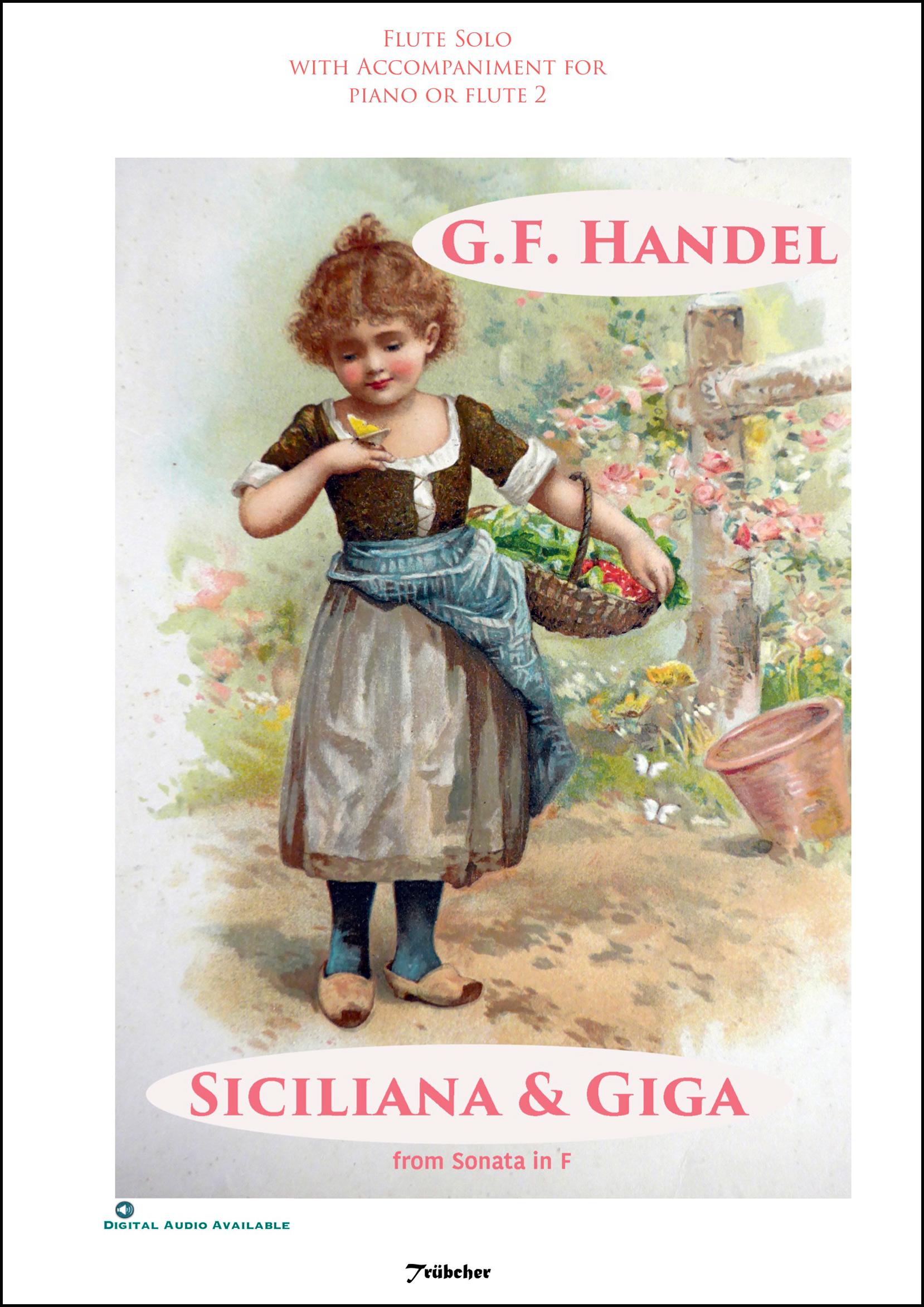This image appears to be a scanned cover of a classical music book or booklet, potentially for flute solo pieces. The top of the white rectangular cover, surrounded by a thin black border, reads "Flute Solo with Accompaniment for Piano or Flute Two" in light pink text. Below this, a central rectangular painting depicts a young girl in a 19th-century-style brown and white dress, complemented by a blue robe or jacket. She has brown hair and is wearing lipstick. In her left hand, she carries a basket containing fruit or berries, while a yellow butterfly perches on her right hand as she gazes at it. The pastoral scene is set in the countryside, featuring a background of a field of flowers, a fence, an empty flower pot, and a wooden cross adorned with flowers to her right. The ground beneath her appears to be white dirt. At the top right in pink text, it says "G.F. Handel," and at the bottom, it reads "Siciliana and Giga from Sonata in F." Additionally, there is a note at the bottom left indicating "Digital Audio Available" with a small speaker symbol above it, and "TriBucker" or "Tribuer" is mentioned in black text at the bottom.